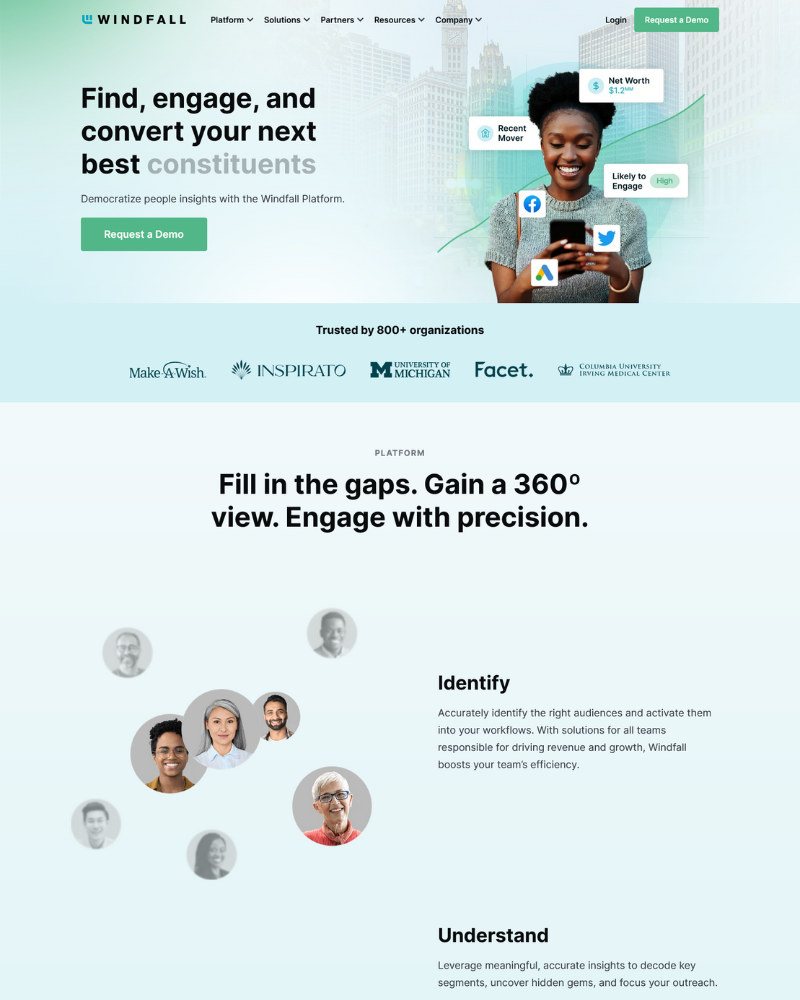The image depicts the homepage of a website, presumably for a company named Windfall. Positioned at the top-left corner of the page is the company's logo or name, "Windfall." Adjacent to this, a horizontal navigation bar features various tabs labeled "Platform," "Solutions," "Partners," "Resource," and "Company." Below this header section, the page is divided into two main sections. On the right side, there is an image of a person using a phone, likely to imply real-world application or user engagement. On the left, bold text reads, "Find, engage and convert your next best constituents," suggesting a focus on customer or client management. This message is complemented by an additional description, which highlights the value of using people insights derived from the Windfall platform. Lastly, a prominent green button labeled "Request a Demo" invites users to explore the platform's capabilities further.